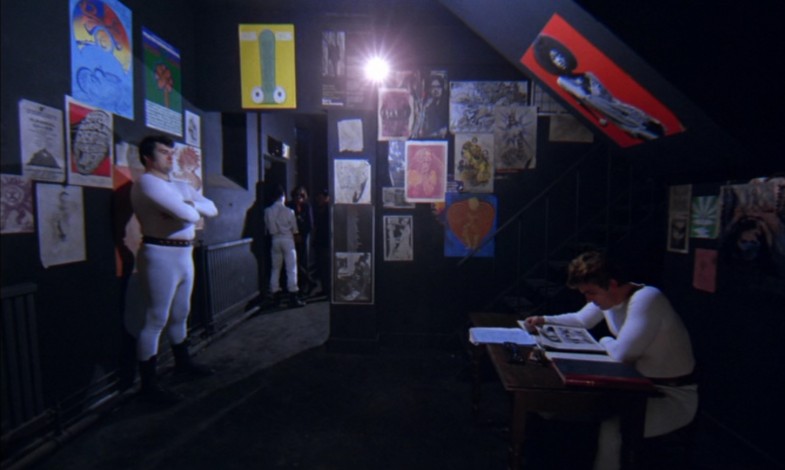In this image, which appears to be a screenshot from a movie or show, we see the interior of a very dark room with nearly black walls adorned with an eclectic array of overlapping posters of various sizes and subjects. On the front wall, a small light fixture shines with white light, illuminating part of the scene. 

To the right, a man with brown hair, dressed in white clothes, is sitting at a small desk with a book open in front of him. He seems to be reading intently. On the left side of the image stands another man, also dressed in white but distinguished by a black belt around his waist and wearing tight gray pants with black boots. With his arms folded across his chest, he has short black hair and appears to be deeply engrossed in his surroundings or possibly in a conversation.

In the background through a door on the front wall, a hallway is visible, showing more people standing, suggesting this room is part of a larger house. The image is horizontally aligned and has a dark, somewhat blurry quality, adding to the scene's mysterious atmosphere.